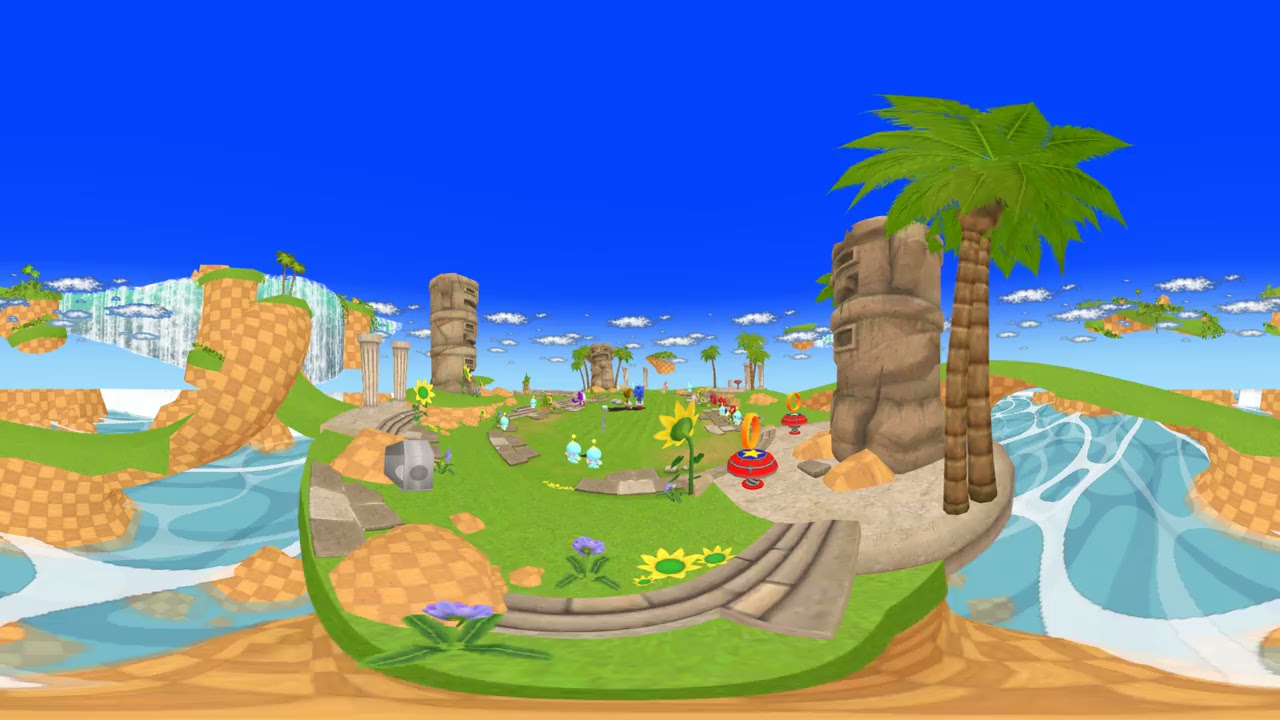The vibrant cartoon game image features a central grassed area with a variety of whimsical elements and potential gameplay features. The bright blue sky is adorned with white clouds, while water bodies flanked by palm trees are visible on both the left and right sides of the image. Two-tiered forts, sunflowers, and blue cartoon creatures with yellow antennae populate the grassy expanse. Purple flowers, possibly lilacs, add a splash of color to the scene.

A fascinating checkered pattern of dark and light orange is seen on land formations, evoking a racetrack or game board look, possibly for placing game pieces. Red springs topped with blue disks and yellow stars hint at interactive game mechanics. In the distance, iconic figures resembling Sonic the Hedgehog and Tails lend a playful, familiar touch to the environment. Hoops to jump through and towering coliseums in the background suggest an exciting and dynamic gameplay experience, enhanced by the twisted, VR-like perspective that warps and bends the landscape, making it visually engaging and immersive.